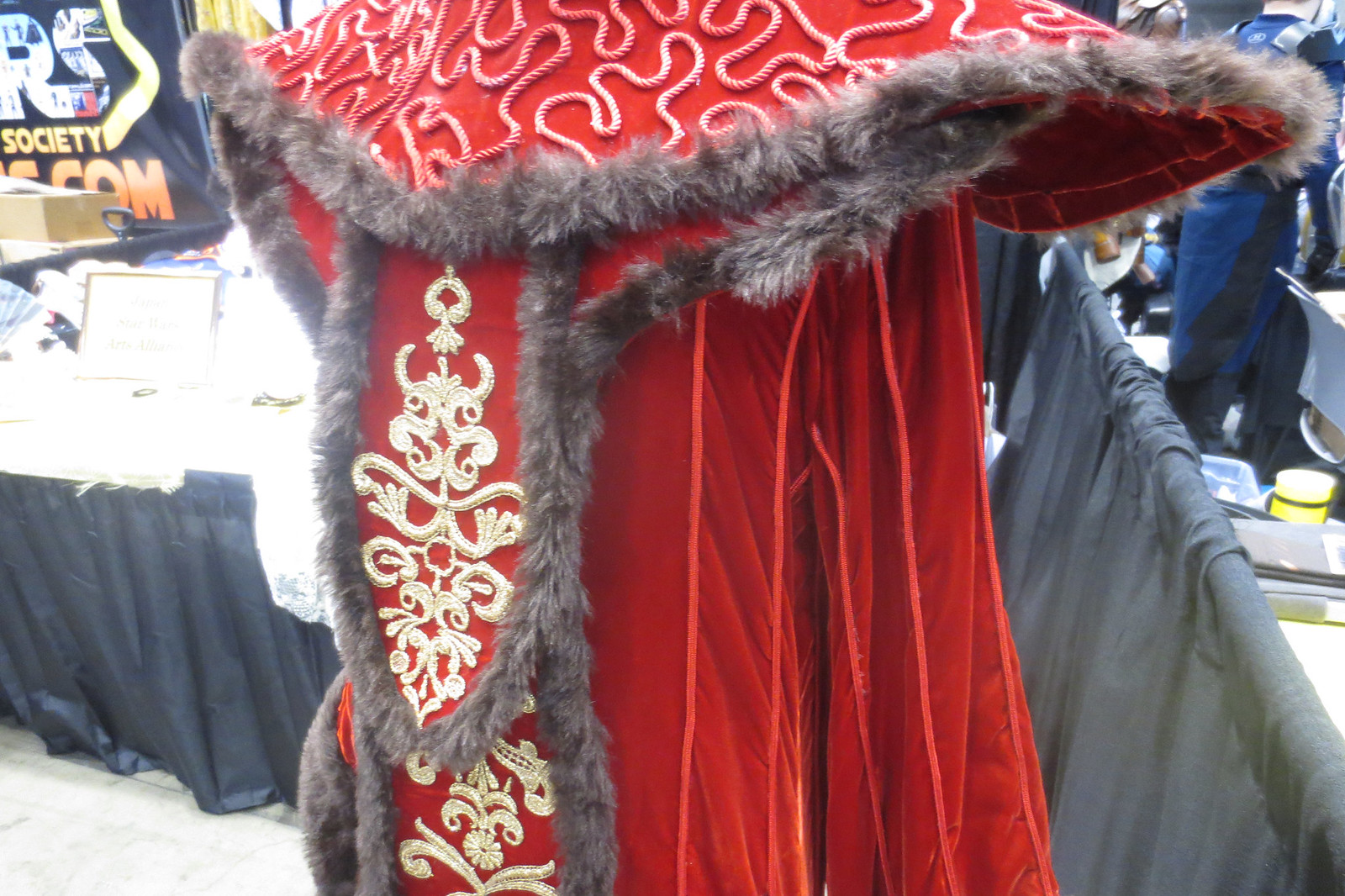The full-color photograph showcases the back of an elaborate costume, which appears to be designed for an event, possibly a convention such as a Comic Con. The costume resembles attire from an Asian movie or anime, characterized by intricate and ornate detailing. It is primarily dark red, accentuated with brighter red stripes on the right side and down the arm. The costume features a cape or shoulder pads lined with fur, and additional material trailing down the back, also fur-lined. Heavy rope embroidery adorns the outfit, with squiggly designs at the top and geometric patterns along the back. The background reveals display tables and a partially visible booth, with a sign reading "RS Society Comm" in the upper left-hand corner, reminiscent of the Star Wars logo, reinforcing the convention-like setting.